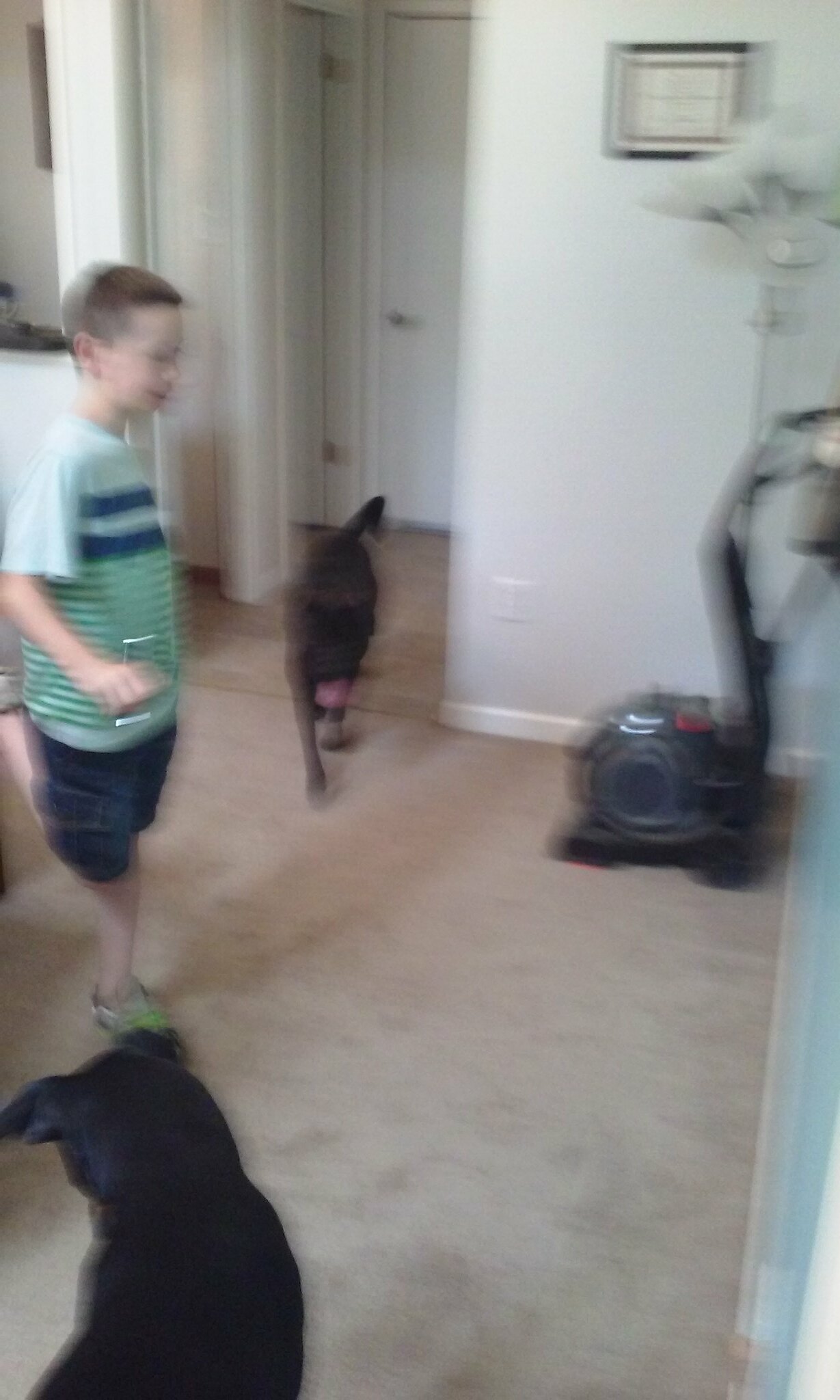In a cozy living room with a cream, almost tan, carpet, a young boy, approximately 8 to 10 years old, stands confidently. A hallway with several doors is visible behind him, providing a glimpse into the adjacent spaces. On the upper right corner of the image, a deep cleaning carpet vacuum stands next to a gooseneck lamp with multiple white plastic lamp heads. Above them, a framed professional degree or diploma in a black plastic frame hangs prominently on the wall.

The boy, who has a short black buzzcut and white complexion, wears a distinctive green-striped t-shirt featuring broad white sections with two big blue stripes and green stripes extending to the bottom. He pairs this with navy blue cargo shorts. In his right hand, he appears to be holding a cell phone, though the object's details are not entirely clear. With his weight balanced on his left leg, his right leg is playfully bent behind him. His outfit is completed with dark navy blue and white sneakers featuring vibrant lime green laces.

Accompanying the boy are two black dogs. The first, possibly an Akita mix weighing around 60-70 pounds, stands to his right. Its pointed ears and curled tail give it a distinctive look, and it appears to be panting, although the photo's slight blur makes it difficult to discern exact details. The second dog, positioned in the lower left corner of the image, has a similar breed appearance. This dog also has pointed ears with slightly floppy tips and is captured in a downward-looking posture, gazing at the floor.